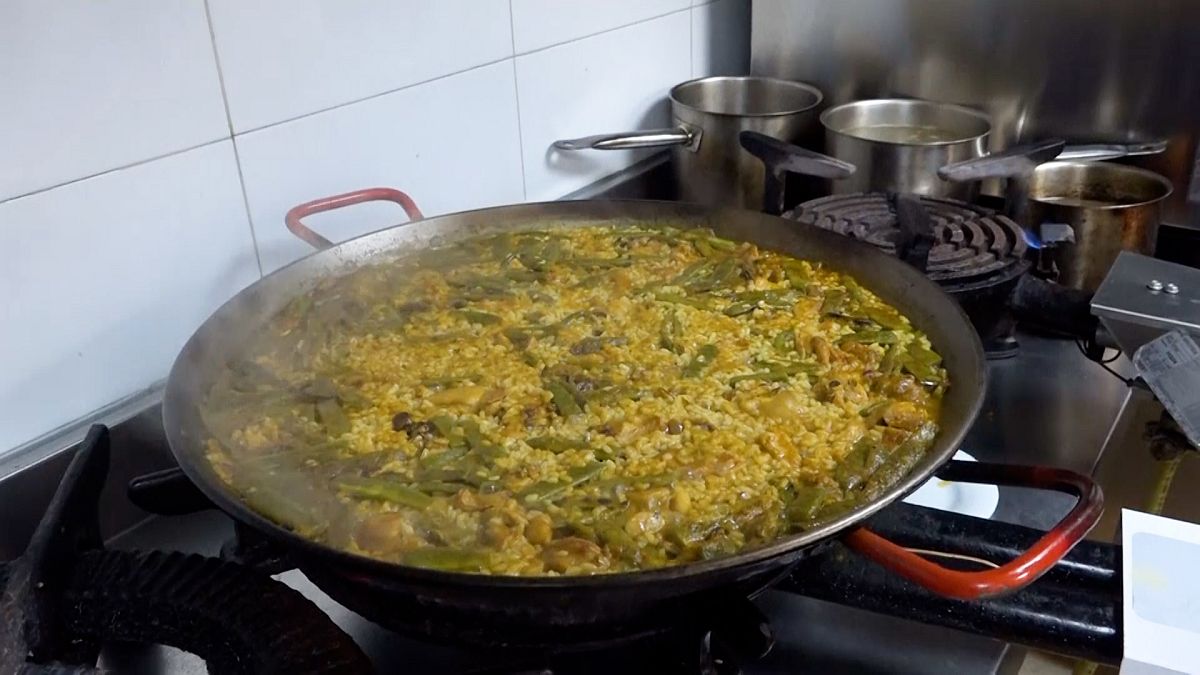The photograph captures a detailed kitchen scene with a focus on a large silver wok with two striking red handles, centrally positioned on a black electric stove. The stove itself appears dark in color, possibly black or dark silver, surrounded by a backdrop of pristine white tile. Adjacent to the wok, there are three additional metal pots, some seemingly containing liquids. In the upper right corner of the image, there's a glimpse of a stainless steel appliance, likely a refrigerator. The wok is filled with a mixed dish of what appears to be fried rice or couscous, featuring a blend of vibrant green vegetables such as green peppers, snow peas, or green beans. Accompanying the vegetables are chunks of brownish meat, possibly pork or mushrooms, all coated in a tan-colored sauce. The well-cooked dish in the wok suggests a savory and tender texture, harmonized by the surrounding kitchen elements.